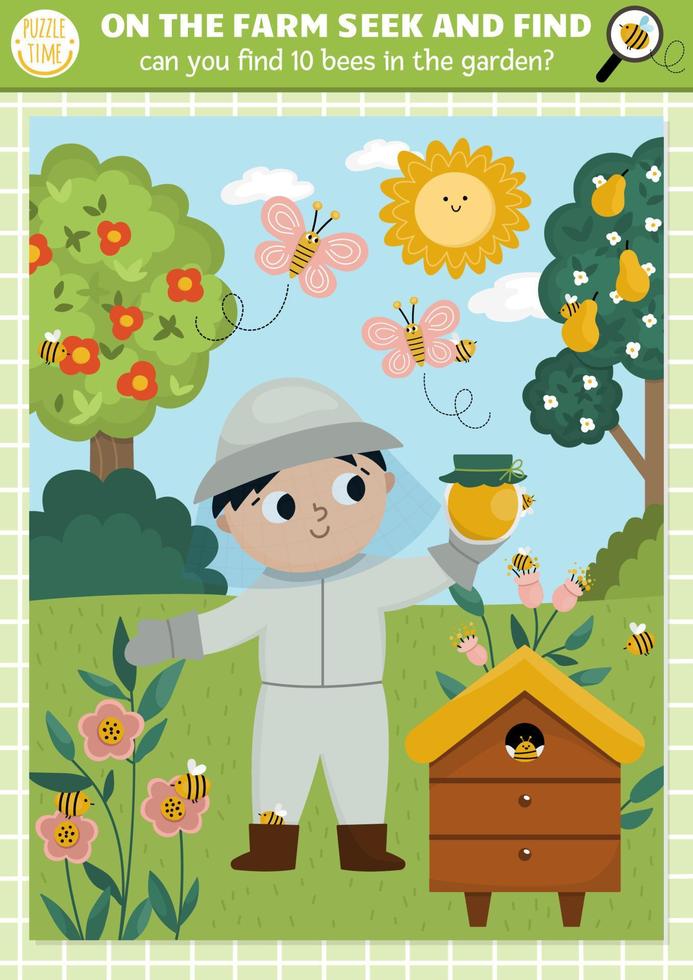The image is a colorful, cartoon-style scene that resembles a page from a children’s activity book titled "On the Farm, Seek and Find" by Puzzle Time. Set against a gradient green border background with a blue sky, the challenge asks viewers to find ten bees scattered throughout a vibrant garden. The title is displayed in white letters at the top, alongside a magnifying glass showing a stylized bee and the Puzzle Time logo.

In the foreground, a young beekeeping boy stands beside a beehive, holding an unusual, cloth-topped jar of honey. He is dressed in a beekeeping suit with a distinctive rounded top hat. Surrounding him are blooming flowers with bees buzzing in and out, along with butterflies and bushes. To the left of the boy, a flowering tree stands, while a pear tree is visible on the right.

The bees to be found are hidden in various places: two in the flowers in the front, one in the beehive, two around the flowers near it, one near the jar of honey, one behind a pear, one near a butterfly, and one on a flower in the flowering tree.